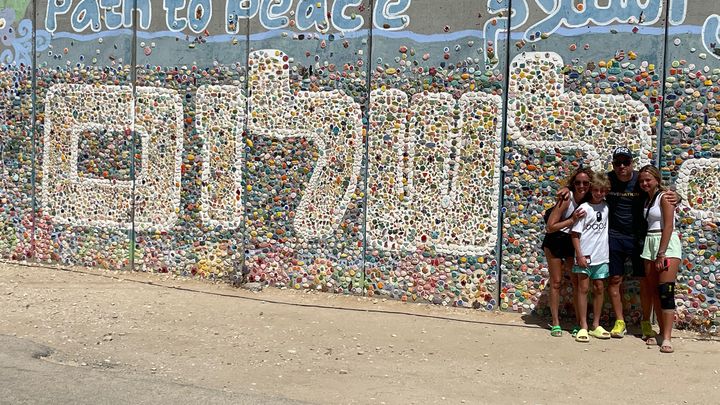In this outdoor family photo, four family members stand smiling in front of an intricately designed wall adorned with colorful stones, shells, and a mural with a blue octopus in the top left corner. Above the mural are the words "Path to Peace," along with some characters that appear to be from an Eastern Asian language. The family consists of a father, mother, young son, and teenage daughter, all dressed in casual summer attire, including t-shirts, shorts, and sandals. The father, on the right side of the image next to his young daughter who sports a knee brace and green shorts, is wearing dark clothing, bright yellow shoes, a hat, and sunglasses. The young son, positioned between the mother and father, sports blue shorts and a white t-shirt, and has blonde hair. The mother, standing on the far left, wears green sandals, black shorts, a white tank top, and sunglasses, with a purse visible behind her shoulder. They stand on a gravelly path, posing happily in front of the vibrant and artistic backdrop.